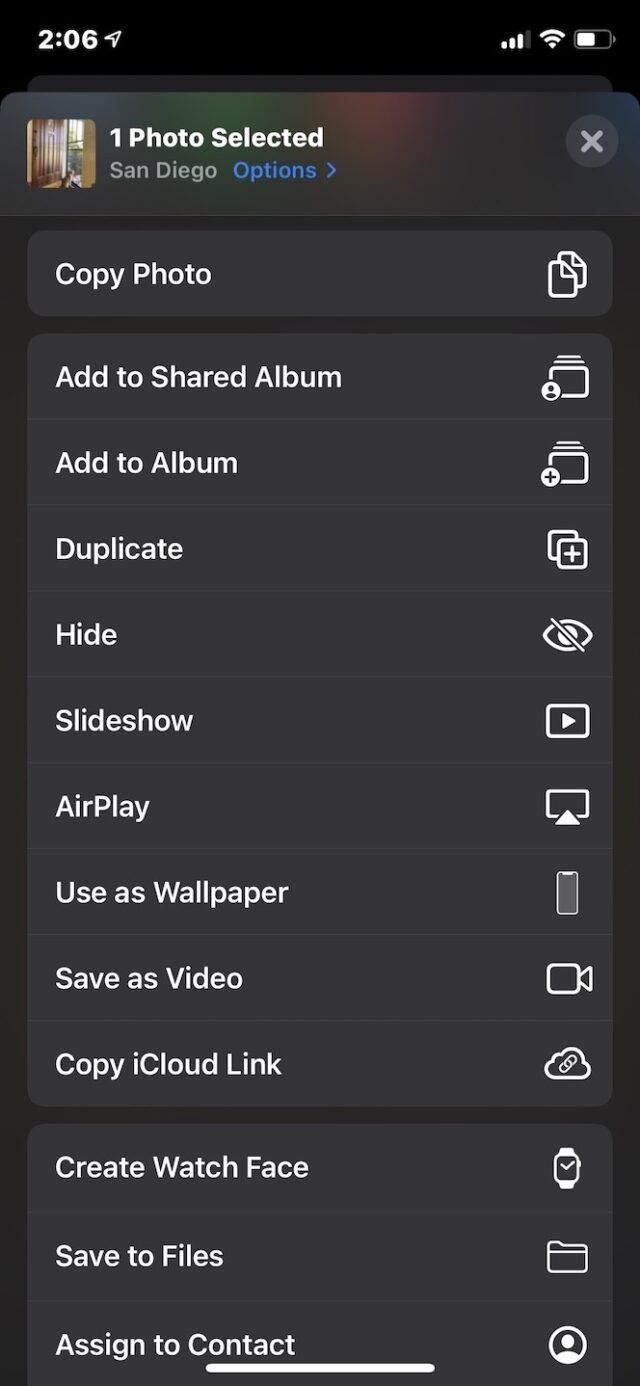This image is a screenshot captured from a cell phone. The entire background is predominantly black. At the top left corner, the screen displays the time as "2:06" along with an icon resembling a small paper airplane. 

Towards the upper middle section, there are slight reflections of shiny red and green, possibly caused by a reflection during the photo capture. On the top right, indicators show that the battery is approximately two-thirds charged, Wi-Fi is connected, and the signal bars are visible.

The screen indicates "1 Photo Selected" with the location marked as "San Diego". Beneath that, the options menu appears. A tiny thumbnail of the selected photo is situated on the left. Various actions are listed in white text, including:

- "Copy Photo"
- "Add to Shared Album"
- "Add to Album"
- "Duplicate"
- "Hide"
- "Slideshow"
- "AirPlay"
- "Use as Wallpaper"
- "Save as Video"
- "Copy iCloud Link"

A thin black line separates the options, leading to additional actions such as:

- "Create Watch Face"
- "Save to Files"
- "Assign to Contact"